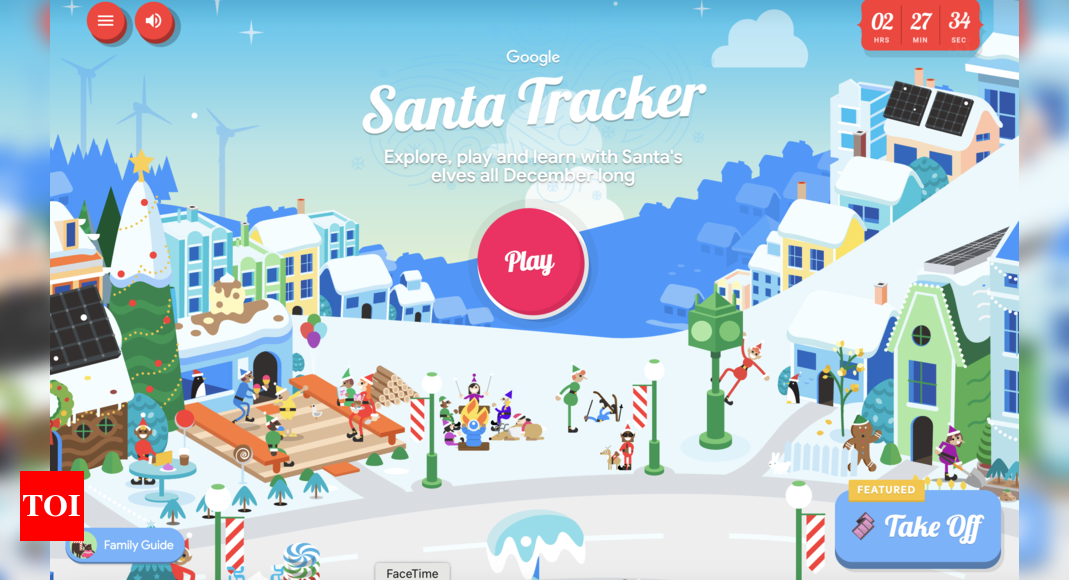This image showcases a Google-sponsored page prominently featuring the "Google Santa Tracker." At the center, the text "Google Santa Tracker" is displayed in white, accompanied by the tagline, "Explore, play, and learn with Santa's elves all December long." Below this, a red circular play button with the word "Play" scripted in white cursive invites interaction.

In the upper left corner, there are two round red buttons: one is a list icon, and the other is a speaker icon. The top right corner displays a countdown timer showing 2 hours, 27 minutes, and 34 seconds remaining.

The background depicts a festive town scene blanketed in snow, with houses lining the street. At the bottom left, there is a "Family Guide" button, and beside it, a label marked "To I." On the right side, positioned under a "Featured" tab, a button labeled "Take Off" is visible. Scattered throughout the scene are small groups of people enjoying the snowy festivities, adding to the holiday ambiance.